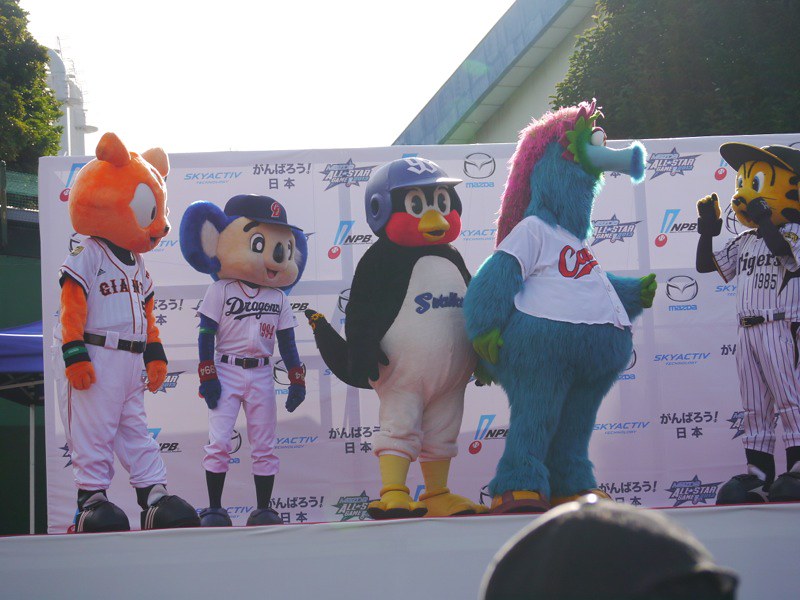The image shows a brightly sunlit day with a light blue or white sky and a few trees and a blue-and-white roof overhang in the background. A large, white stage takes up the center of the picture, with a white banner behind it featuring logos and texts such as "All-Star Games," "MPB," Mazda, SkyActive, and some Asian writing. At the bottom right of the image, the front edge of the stage is visible, and a black hat can be seen protruding from it.

On the stage, five mascots are lined up from left to right in front of the banner. The first mascot on the left is a brown or orange mouse-like character wearing a white Giants uniform with black shoes and arms at its side. Next is a shorter, blue-and-white mouse mascot with big blue ears, a blue hat with a red emblem, black socks, and blue shoes. It wears a white uniform labeled "Dragons." 

In the middle stands a penguin mascot with a red area around its mouth, black arms and back, a white chest, yellow feet, and a yellow beak. It sports a blue helmet. To its right is a fuzzy, blue mascot with a long neck, pink hair, green face, and a distinctive, tuba-like nose, resembling the Philly Phanatic. It has a white shirt with red letters partially visible.

The final mascot, on the far right, is a tiger with a black-and-yellow face, black markings, and a white striped baseball uniform reading "Tigers 1985." The tiger has its hands raised near its face and is facing the other mascots. The scene includes glimpses of buildings and the skyline in the background.